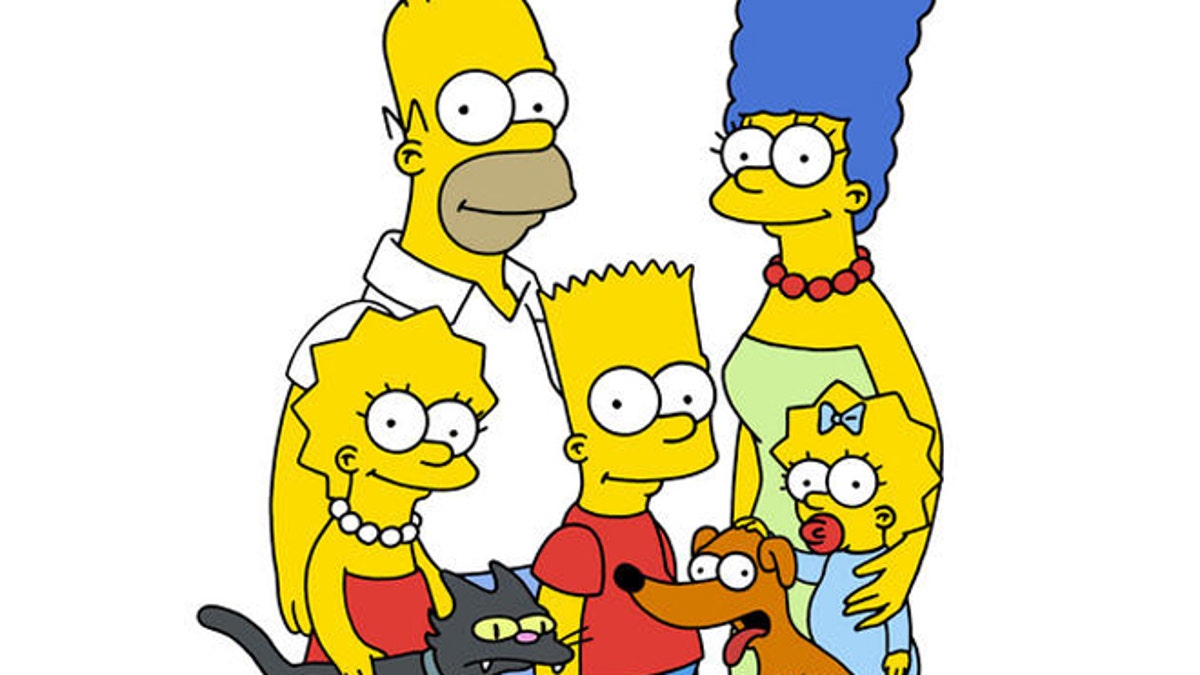This image depicts the iconic Simpsons family from the long-running animated series "The Simpsons." The family, set against a plain white background, includes Homer, Marge, Bart, Lisa, and Maggie, all with their characteristic yellow skin. Homer, the bald father with an oval-shaped head and an "M"-shaped hairline, is dressed in a white shirt and has a notable beer gut. Standing beside him is Marge, the mother, recognizable by her towering blue hair in an afro shape and her green dress paired with a red pearl necklace. 

In the bottom left, Lisa, their eldest daughter, is seen wearing a red dress and white pearl necklace, and she's petting their black cat, which sports a blue collar. Bart, the mischievous son, stands at the center of the picture in his signature red shirt and blue shorts, with his spiky hair adding to his distinct look. Next to Bart, in the bottom right, is their dog, Santa’s Little Helper, a brown dog with a black olive-shaped nose, crooked googly eyes, and its tongue playfully hanging out. Finally, Maggie, the baby, to the right of Bart, is adorned in a pale blue onesie, a red pacifier in her mouth, and a blue bow in her hair. All family members, except for Marge, have white eyes with single black dots, capturing their classic animated expressions.